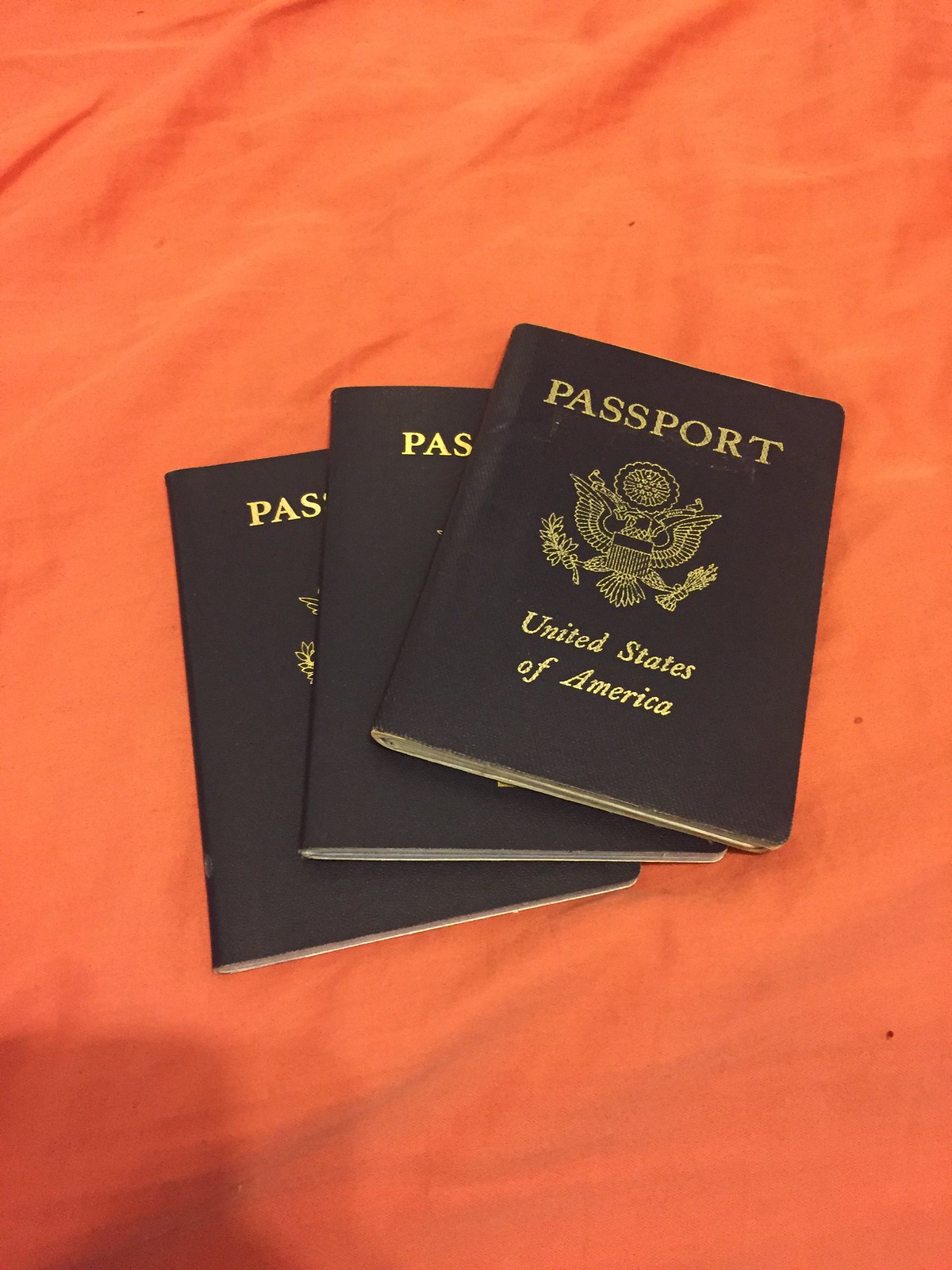This photograph showcases a detailed arrangement of three black American passports, fanned out from left to right, centered on a wrinkled orange cloth that fills the entire background. The passports, made of what appears to be leather, each feature gold embossed text and imagery. At the top, the word "PASSPORT" is stamped in capital letters, and at the bottom, "United States of America" is inscribed. The central passport's front cover is fully visible, while the others have portions of their text obscured. A gold-embossed eagle, holding branches in its talons, is prominently displayed on the cover. A shadow, likely cast by the camera, is noticeable in the bottom left corner, adding a subtle depth to the image.